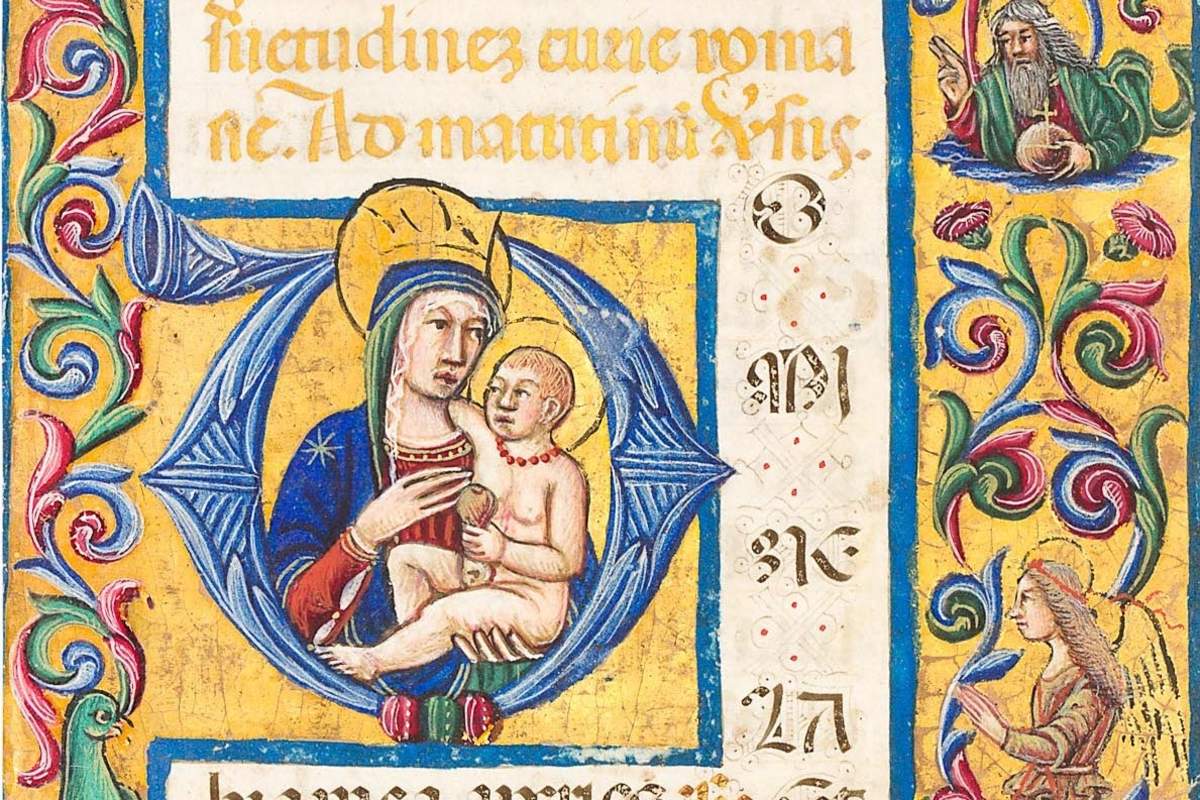This highly detailed image features an intricate, up-close view of a medieval manuscript, seemingly written in Latin. At the center, within a large, ornamental letter "O," sits the Virgin Mary adorned in a blue robe, holding the baby Jesus. Both figures are crowned with radiant halos, emphasizing their sanctity. The manuscript also depicts several other Christian figures. To the bottom right, there's an angel, although the paint is chipped and worn. Along the right side of the manuscript runs a vertical golden stripe decorated with foliage and flowers in red, blue, and green hues. This stripe includes a figure with long, light-colored hair and a beard, dressed in a green robe and wearing a crucifix necklace. The figure, possibly a priest or a saint, holds a globe topped with a cross. Surrounding Mary and Jesus, and spread throughout the design, are various decorative elements such as sideways orbs, peacock-like birds, and feather motifs. The manuscript exhibits considerable age and historical richness, with its text being either in a foreign script or a highly stylized, illegible form.